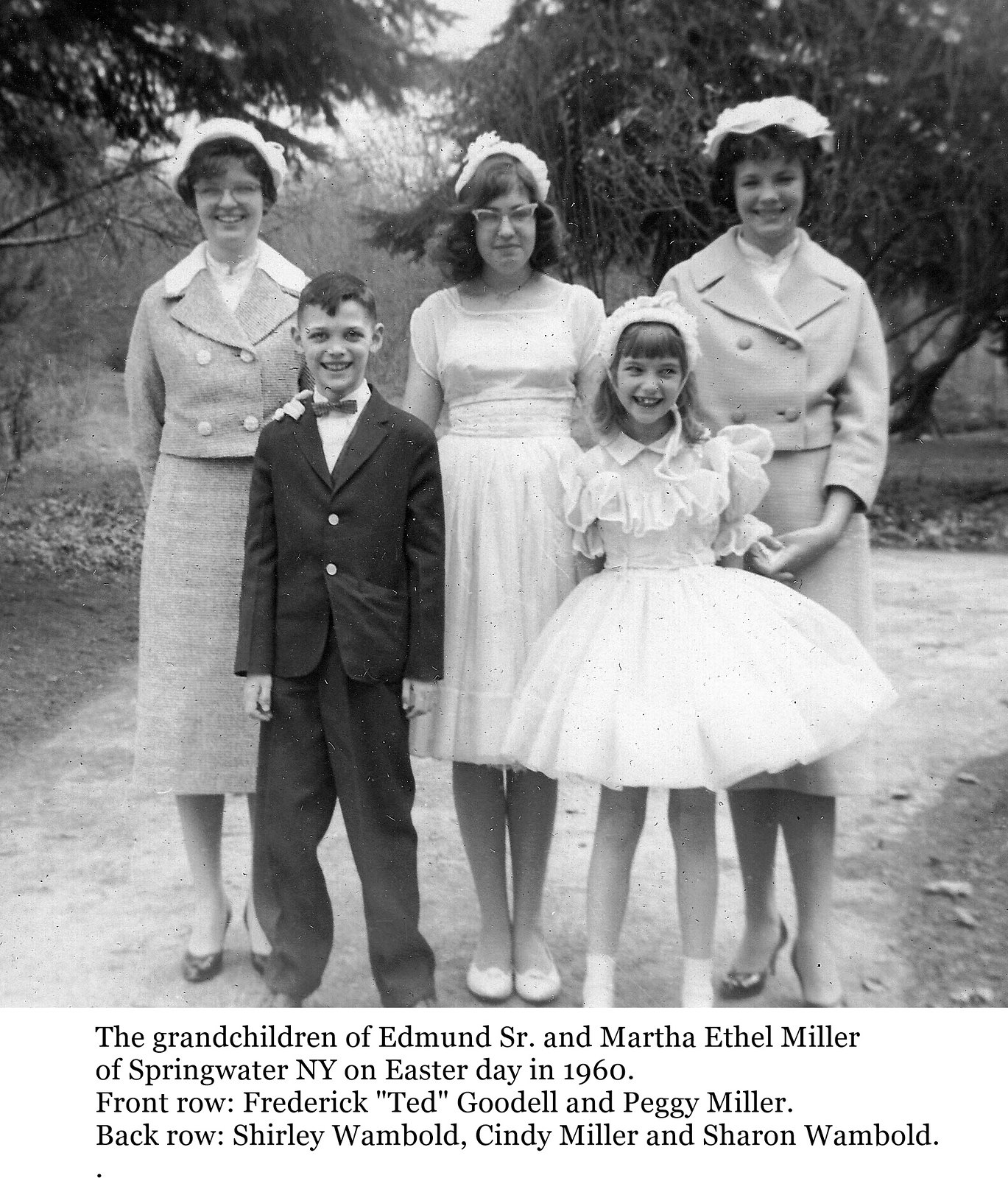This black-and-white photo, taken on Easter Day in 1960, captures the grandchildren of Edmund Senior and Martha Ethel Miller of Springwater, New York. Set against a backdrop of trees, this daytime image includes five individuals, with the three women standing in the back and two children in the front. In the front row, on the left, Frederick Ted Goodell wears a dark tuxedo with a bowtie and white collared shirt, his hair cut short. Beside him stands Peggy Miller, around eight or nine years old, dressed in a large, frilly tutu-like white dress. 

In the back from left to right, are Shirley Wambold, Cindy Miller, and Sharon Wambold. All three women don vintage outfits, complete with short white hats. Shirley, on the left, wears a suit-type ensemble with a skirt that falls below her knees. Cindy, in the center, has shoulder-length dark hair and wears a white dress that ends just above her knees, complemented by cat-eye glasses. Sharon, positioned on the right, wears an overcoat with large collars and a belt. The caption at the bottom of the photo reads: "The grandchildren of Edmund Sr. and Martha Ethel Miller of Springwater, New York on Easter Day in 1960."